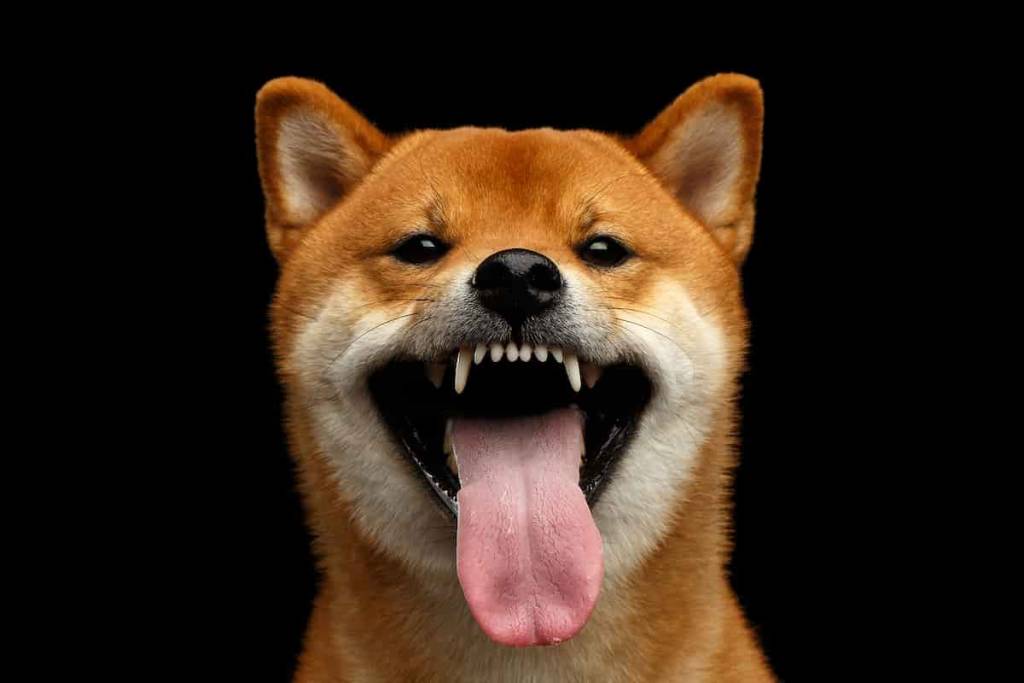This photograph captures a Shiba Inu, medium-sized and fawn-colored, giving the impression of a broad smile directly at the camera. Its mouth is wide open, displaying a healthy set of white teeth and a pink tongue hanging out. The dog's face is adorned with distinctive white markings around the muzzle and ears, complementing the neat and well-groomed brown fur. Its eyes are dark and almond-shaped, and it has a black nose. The background is a pitch-black void, emphasizing the vibrant and contrasting colors of the dog's coat and features. The entire composition focuses on the dog’s expressive and joyful demeanor, making it appear as though it's genuinely smiling.